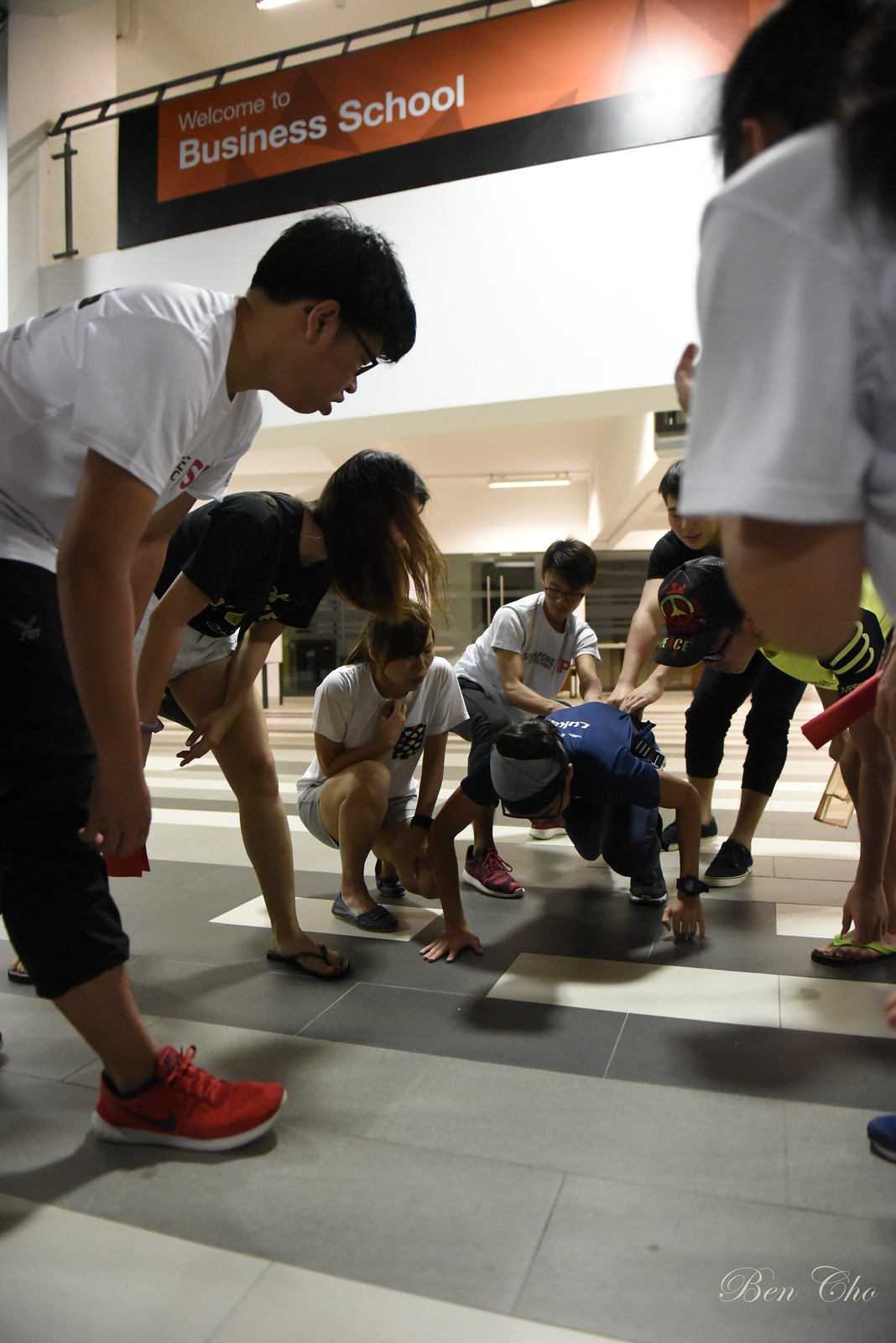In this image, a group of teenagers, both young men and young women, are gathered in an auditorium with a floor of black and white tiles. The room is brightly lit with white walls, and a prominent banner overhead reads "Welcome to Business School" in white letters against a red and black background. At the center of the scene, a person in a blue t-shirt is on the ground in a plank or push-up position, with bent elbows and hands on the floor. There is some ambiguity about whether they are doing push-ups or getting up from the ground. Surrounding them, other teenagers are either watching intently or interacting with the person on the ground, possibly placing their hands on their back, which might be to add tension or pressure. Notable figures include a boy with black hair, red shoes, glasses, and a white t-shirt, and a girl with a ponytail and a white shirt. The setting suggests an informal activity or exercise, typical of group dynamics among young people in a school setting.